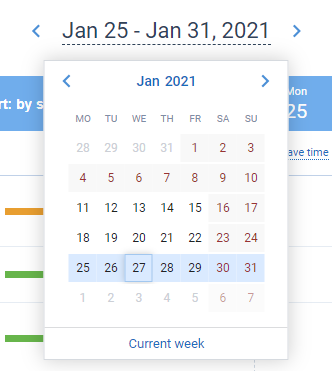The visual representation is a detailed timeline calendar for January 2021. 

In the top-left, a blue arrow marks the beginning of the timeline, followed by the text "January 25th - January 31st, 2021," with another blue arrow on the right to indicate the timeline's extent. Below that, there are underlined dashes likely serving as dividers or indicators of segments.

At the center, a large window displays the calendar for January 2021. The top-left and top-right corners of this window have blue arrows, framing the central text that reads "January 2021". 

The calendar grid follows the standard week format, starting from Monday and ending on Sunday. The days are laid out numerically from the 20th to the 24th in the first week, and from the 25th to the 31st in the second week. The calendar continues to show the first week of February 2021 with dates from the 1st to the 7th.

Highlighted within the calendar, a blue bar encompasses the dates from the 25th to the 31st, denoting the current week. Below this, there is a label indicating "current week" in blue text.

Additional visual elements include a segmented bar at the bottom comprising sections of different colors: an orange bar followed by two green progress bars, which likely represent different phases or statuses over the given timeline.